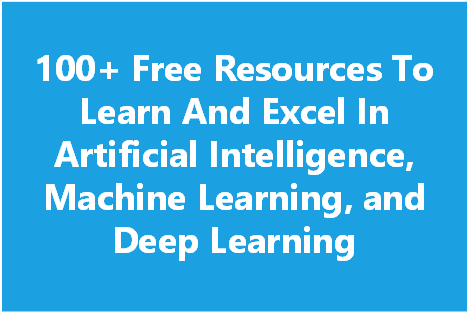Detailed Caption: 

An informational poster showcasing "100+ Free Resources to Learn and Excel in Artificial Intelligence, Machine Learning, and Deep Learning." The text is presented in crisp white letters against a vibrant blue background. The title is prominently displayed, emphasizing the abundance of free educational materials available for those interested in advancing their knowledge and skills in these cutting-edge technological fields. The overall design is clean and professional, making it easy to read and appealing to the audience.